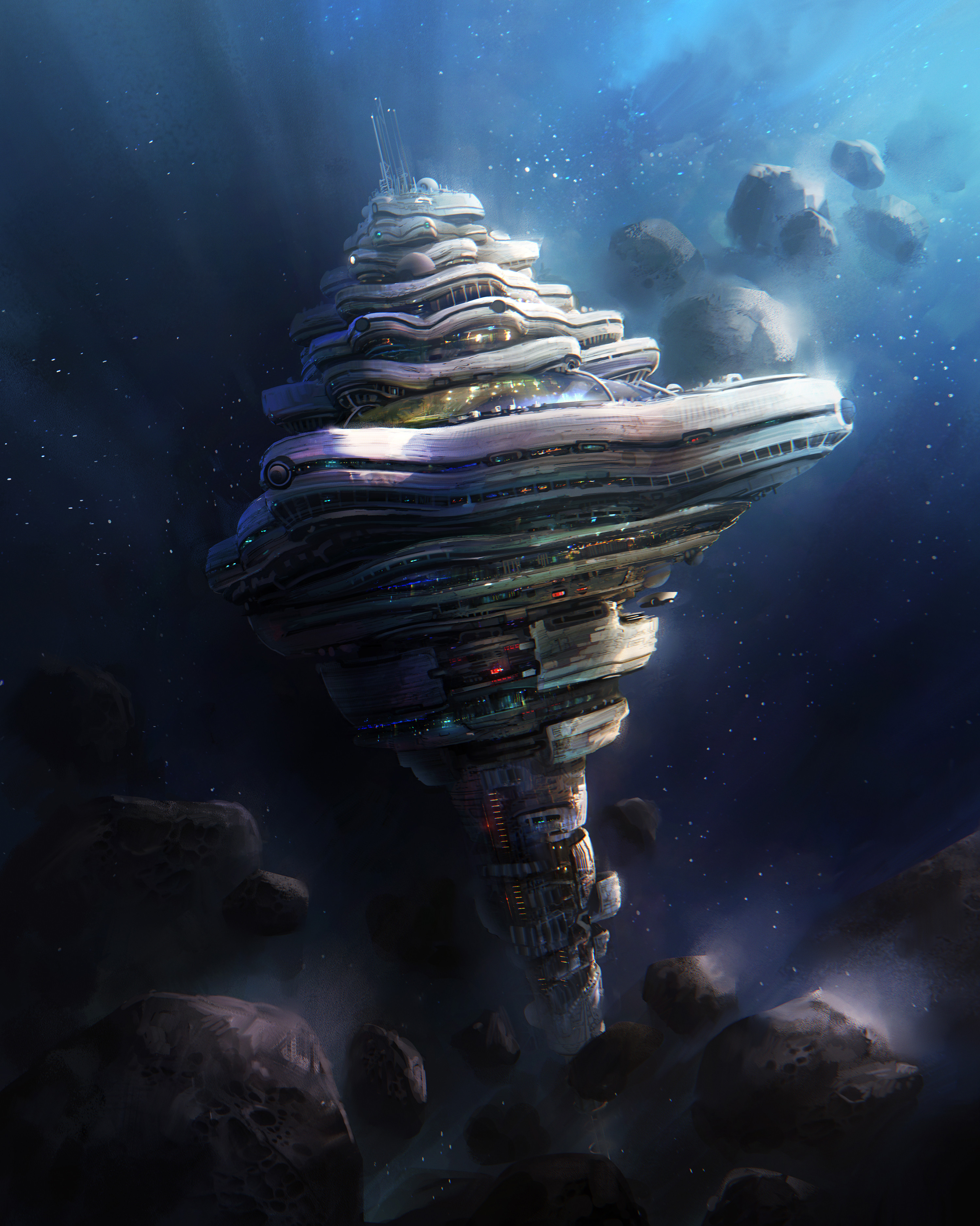This digital artwork depicts a towering, cylindrical space station floating in the depths of outer space, dominated by shades of blue. The station, which resembles a series of interconnected shells or decks, is adorned with numerous antennas or signal lines on its uppermost section. Brilliant lights of red, green, and blue illuminate various parts of the structure, adding a stark contrast to the surrounding darkness. The scene is enriched with floating asteroids above and below the station, creating a dynamic sense of motion. Distant stars sprinkle the background, enhancing the sci-fi atmosphere of this immersive, computer-generated image. The dark expanse around the station makes the details pop, emphasizing both the isolation and the grandeur of this otherworldly setting.